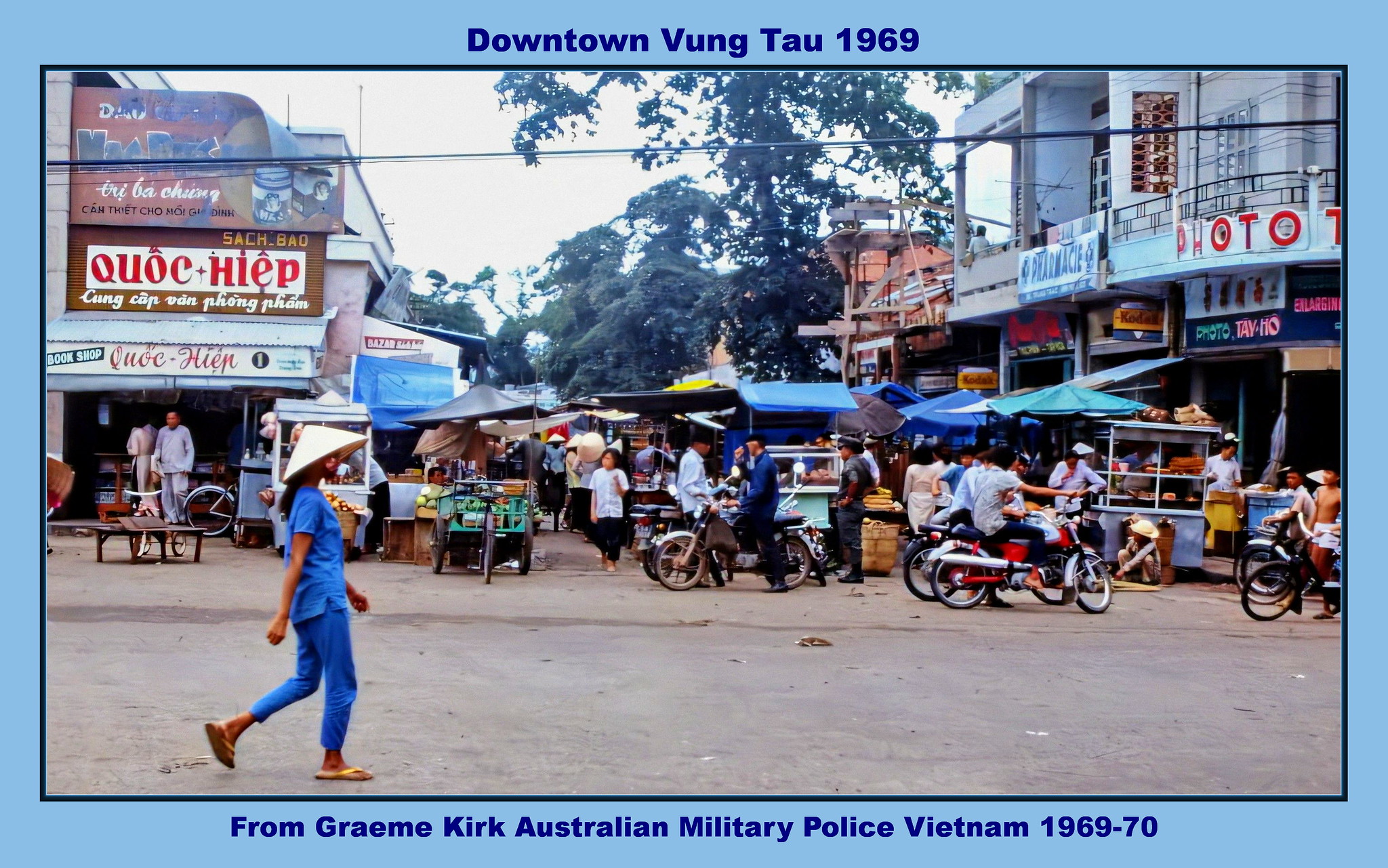This photograph captures a bustling outdoor marketplace in downtown Vung Tau, Vietnam, circa 1969. The scene is vibrant with numerous shops and stands lining the street, each shaded by colorful umbrellas in hues of blue, yellow, green, black, and white. The marketplace is crowded with people, some walking, some riding motorbikes or bicycles. A woman in the foreground stands out, dressed in a blue outfit and wearing a traditional triangular straw hat. The marketplace is flanked by buildings on both sides, and Vietnamese signs are visible throughout the scene. In the distance, a large mountain capped with white snow provides a striking natural backdrop. The photograph is framed with a light blue border, with "Downtown Vung Tau, 1969" inscribed at the top in dark blue text, and "From Graham Kirk, Australian Military Police, Vietnam 1969-70" at the bottom.